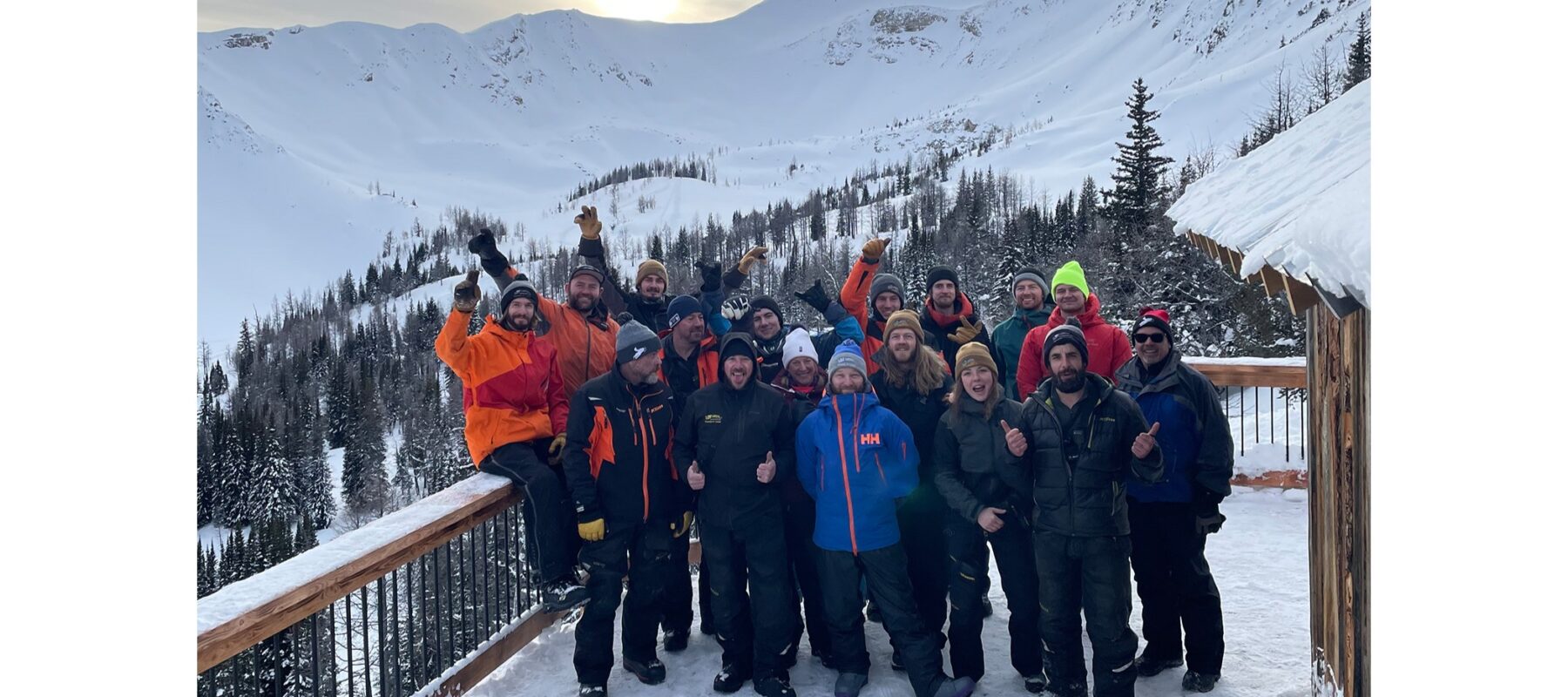In this vibrant color snapshot, a spirited group of 17 outdoor enthusiasts, dressed in insulated winter clothing, stands on the snow-covered wooden deck of a mountain lodge. The scene is set against the backdrop of a snowy mountain valley, with coniferous trees lining the lower slopes and the valley floor. The mountains, dusted in snow, rise majestically in the background as the sun peeks over the ridges, casting a golden hue across the landscape. Among the group, which consists predominantly of men with a few women, three individuals wearing orange and blue jackets sit on the deck railing, their hands raised in exuberant celebration. Knit hats and sunglasses are common accessories, adding to their prepared and festive look. The photographer, positioned above, captures this joyous winter gathering as they revel in the breathtaking natural beauty surrounding them.